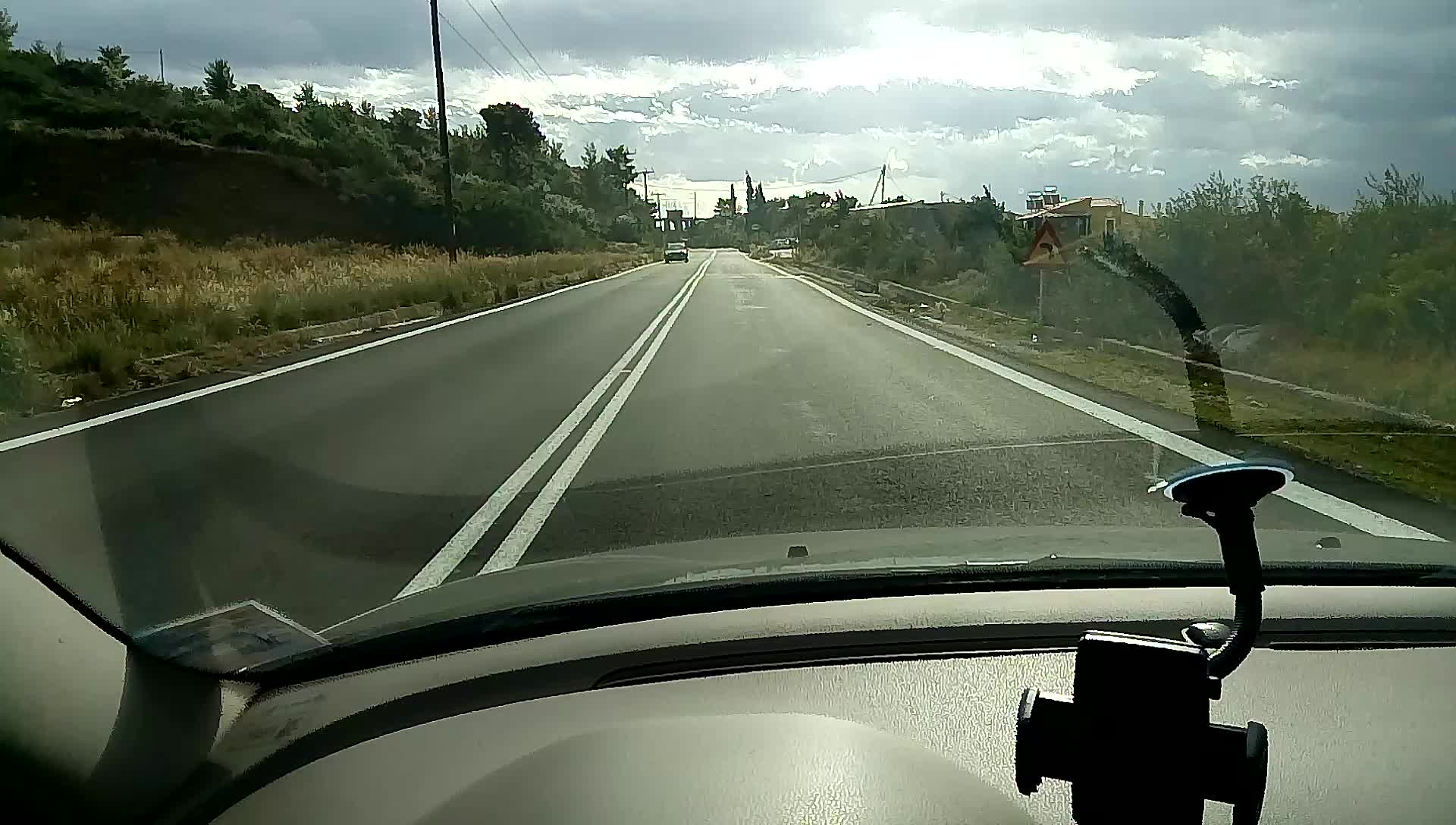This image captures the view from the driver's seat of a vehicle traveling down a two-lane highway. The dashboard of the car is visible in the foreground, featuring a phone holder attached to the windshield. Through the windshield, a two-lane highway stretches ahead with distinct double yellow lines marking the center. On either side of the highway, lush green grass and tall trees line the road, creating a serene, natural border. In the distance, a car is seen approaching from the opposite direction. Further in the background, beyond the trees, utility poles or some tall structures are faintly visible. The sky above is mostly cloudy but allows sunlight to filter through, casting a diffused glow over the scene, adding a touch of warmth and tranquility.